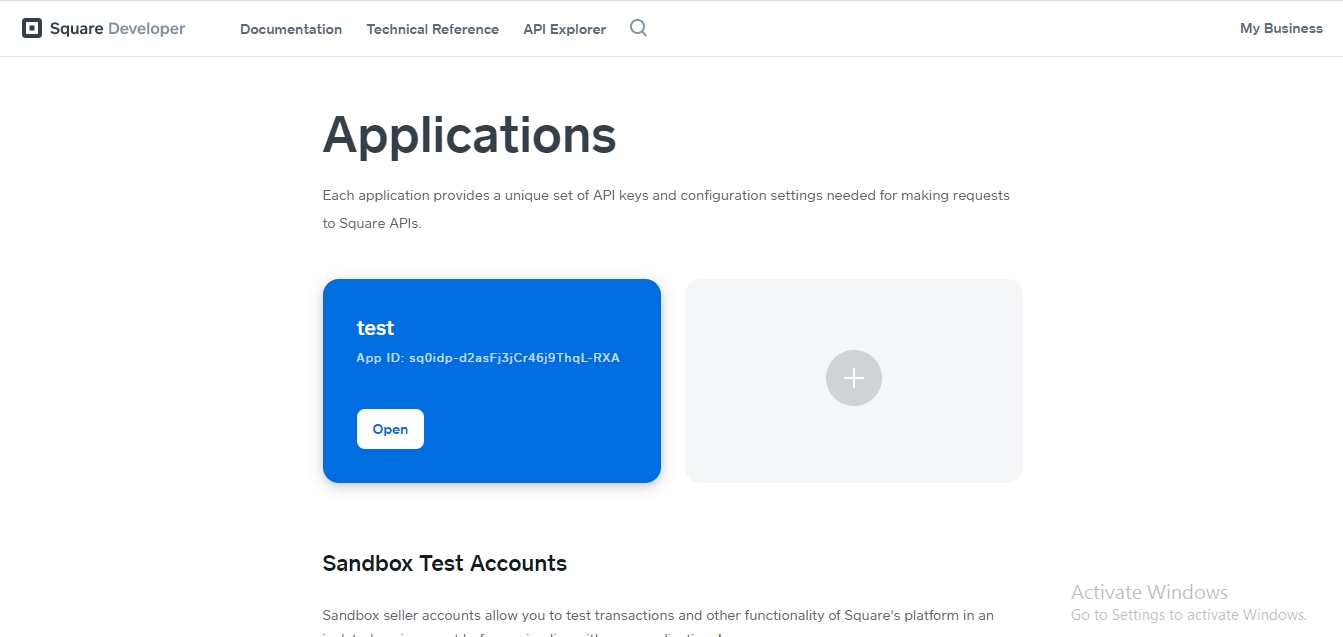This screenshot is from the SquareDeveloper website, showcasing its user interface. In the top left corner, the "SquareDeveloper" logo is prominently displayed. On the same row, towards the center and right section, there are several navigational options listed: "Documentation," "Technical References," "API Explorer," a search bar with a magnifying glass icon, and "My Business." 

The webpage background is white, with the central focal point featuring the title "Applications" in large, bold black text. Directly beneath this title, a smaller line of text explains, "Each application provides a unique set of API keys and configuration settings needed for making requests to Square APIs."

Below this explanatory text are two distinct boxes. The left box is blue and contains a test API ID, represented as a serial number comprising letters and numbers, alongside a white button labeled "Open." The right box is transparent with a white cross icon at its center.

Beneath these boxes, another description titled "Sandbox test accounts" is presented. This section elaborates, "Sandbox seller accounts allow you to test transactions and other functionality of Square's platform."

In the bottom right corner of the screenshot, there is a gray text notification that reads, "Activate Windows. Go to Settings to activate Windows."